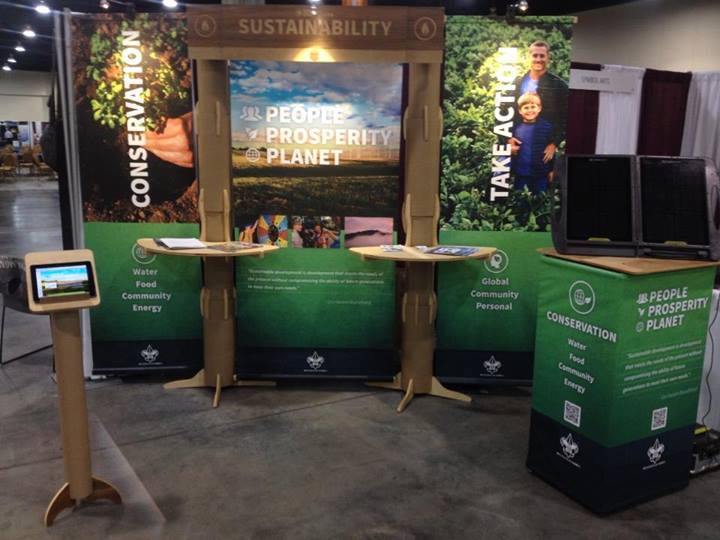The image showcases a detailed setup of a promotional booth at a convention center, distinguished by its emphasis on conservation and sustainability. The booth features a large temporary wall, reminiscent of an open pamphlet, with a vivid green backdrop adorned with tree imagery and greenery. The left panel prominently displays the word "Conservation," accompanied by a human hand holding leafy vegetation. The right panel reads "Take Action" and includes an image of a man and a small blonde boy standing in a lush field, symbolizing family involvement. The center panel features a serene blue sky with clouds, emblazoned with the words “People, Prosperity, Planet” in white text. 

At the bottom of these panels, additional green blocks of information are visible, though partially obscured. Centrally located in front of the wall are two light brown, semi-circle tables covered with literature and pamphlets for visitor interaction, emphasizing topics like water, food, community, energy, and sustainability. To the left of the tables stands a large promotional box reiterating the themes of conservation and wellbeing. Adjacent to the left panel, a sleek stand with a tablet is positioned for digital interaction. Encircling the top of the pamphlet-like wall, a brown archway displays the word "Sustainability." 

The floor is covered with a gray carpet, and in the background, the expansive convention center can be seen, adding context to the booth’s placement within the larger event space. To the right, two large speakers and additional screens provide further engagement opportunities for attendees.